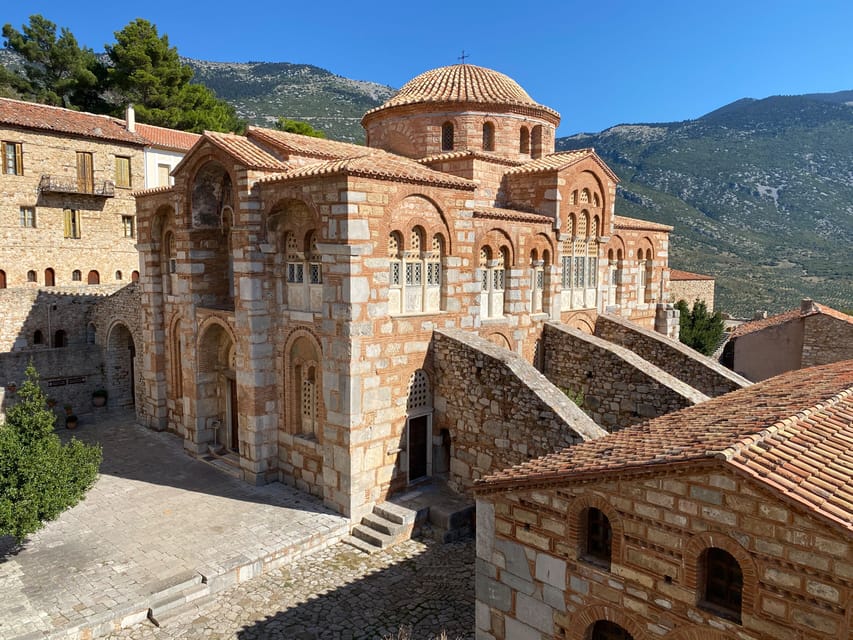Set against a backdrop of hills and majestic mountains, this captivating image captures a cluster of historic buildings that exude an old-world charm. The centerpiece is a two-story edifice with a distinct dome-shaped tower adorned with arched windows. Crafted meticulously from a blend of tan, brown, and white brick and stone, the buildings reflect a bygone era of architectural craftsmanship. The environment looks like a picturesque destination you'd find in a travel magazine, perhaps situated in a country known for its rich historical and cultural heritage. Cobblestone paths lead up to these impressive structures, and although the landscape is sparse with only a few vibrant green trees, the clear blue sky overhead adds a serene touch. Staircases made of the same brick and stone add a layer of grandeur, while balconies accentuate the classic architectural design, suggesting that these might have once been, or still are, elegant homes or possibly even religious buildings.